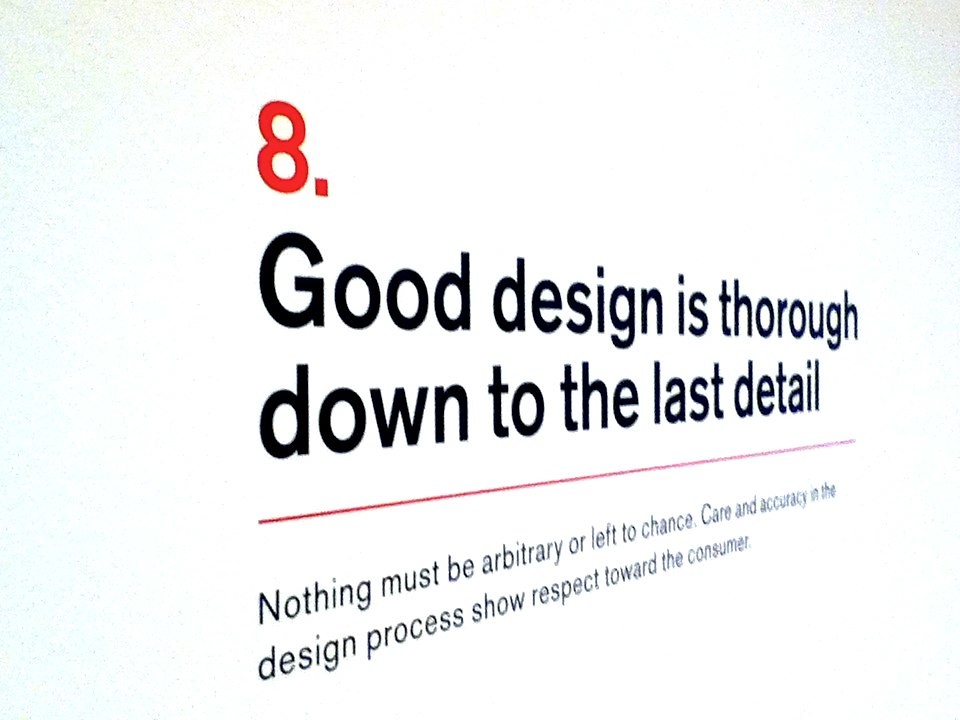The image features a white background with some grainy texture in the upper left and right corners. The main content is presented on a sign or page viewed at an angle, causing the text to appear in a diagonal orientation. Dominating the left side, there is a large red number 8. Just below the number, there is a bold black text that reads, "Good design is thorough down to the last detail." Underneath this text is a thin red line stretching across the width of the text. Below the red line, there is smaller black text which states, "Nothing must be arbitrary or left to chance, care and accuracy in the design process show respect toward the consumer." The text becomes blurrier and harder to read as it stretches toward the right side of the image, which subtly transitions to a light bluish-gray color.